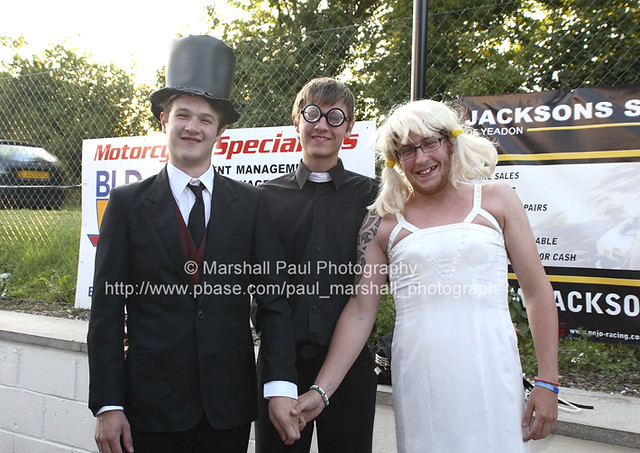This image captures a playful outdoor scene featuring three young men dressed in eclectic costumes. At the center, there's a man dressed like a priest, wearing a black outfit with a white clerical collar and round black-framed glasses. Flanking him on the left is a man in a black suit with a white dress shirt, a burgundy vest, a black tie, and an old-fashioned top hat. He's smiling, adding to the lighthearted atmosphere. On the right, a man in a white wedding dress, adorned with tattoos and bracelets, sports a blonde wig styled in pigtails with yellow ponytail holders. He's holding hands with the man in the suit, suggesting a mock wedding scene. They stand in front of a brick wall and a chain-link fence that features an advertisement, with some grass and the back of a car visible on the left side of the image. The background includes trees and a sky that hints at either sunset or sunrise, given its yellowish hue. The photograph is watermarked with "copyright Marshall Paul photography www.pbase.com/Paul_Marshall_photography" and appears to capture a humorous and staged moment.